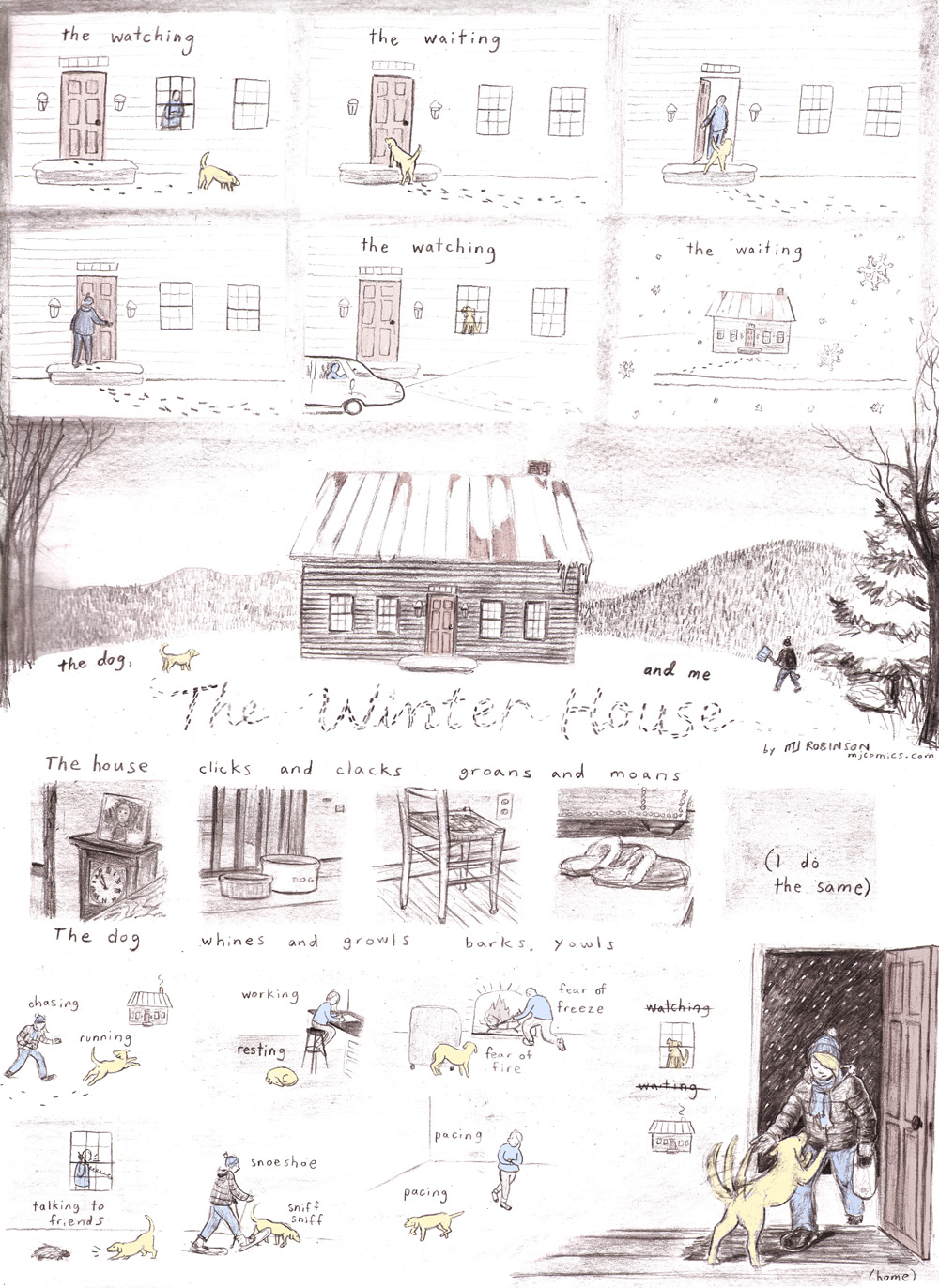The image is a detailed, hand-drawn comic strip resembling a series of crayon illustrations. It comprises around 20 panels depicting a continuous narrative centered around a house and a dog. The first few panels show a sequence where a person is looking out a window at a dog, with captions like "The Watching" and "The Waiting." The story progresses with the person opening and closing the door while the dog waits outside. In the middle of the comic, there is a central panel labeled "The Winter House" showing the exterior of the house with the dog and person outside. Below, a series of panels with captions like "The house clicks and clacks, groans and moans. The dog whines and growls, barks and yowls. I do the same," convey the sounds and activities within the home. The imagery includes the dog running, resting, communicating with friends, and reacting to the environment. Colorful shades of brown, white, black, yellow, gray, blue, and tan accentuate the wintery, outdoor setting. The final panels depict a woman returning home as the dog eagerly wags its tail, completing the heartwarming tale of companionship during winter.